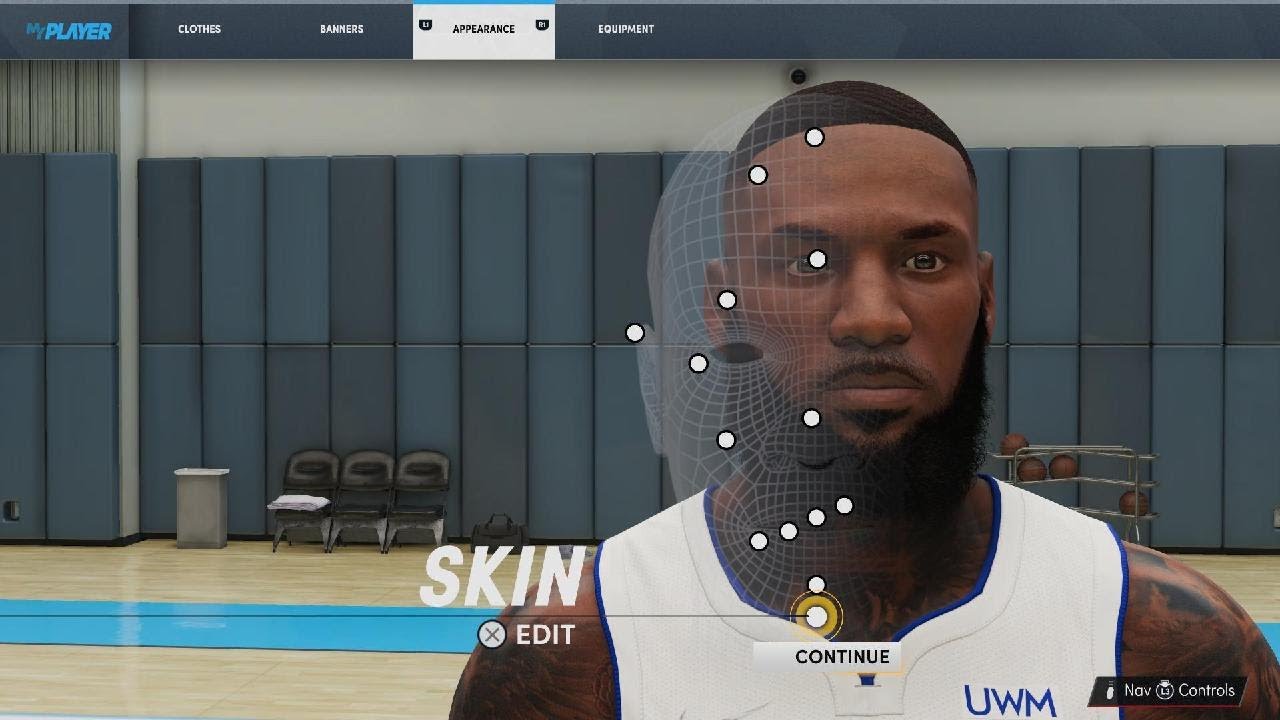In this image, a Black man wearing a white tank top with the letters "UWM" on the left pectoral area is seen. He sports a beard, mustache, and has various tattoos, alongside a very short haircut. The setting appears to be a gymnasium. On the upper edge of the photo, there's a black band with blue text reading "My Player."

The environment includes clothes, banners, and gym equipment, suggesting an athletic setting. The photo also features an X-box icon within a circle and various interface elements. On the bottom right, text reads "Now you controls," indicating an on-screen editing program.

The man's face shows a transparent grid pattern hovering to the right side, with 14 white circular points evenly distributed around it. This suggests that the image is likely part of a facial recognition or skin-editing feature within the software.